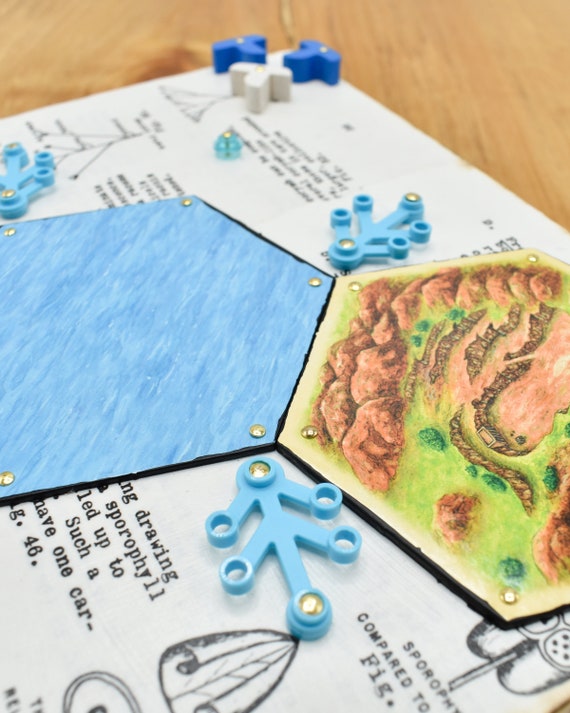The image depicts a close-up of a detailed and intricate setup on a white rectangular board, which appears to be positioned on a brown wooden table. The board is filled with various elements, such as text and decorative items, giving it the appearance of possibly being a scientific diagram or part of a board game. Much of the text on this board is obscured by two main panel-like pieces. One of these panels is a blue hexagon, while the other features an illustrative scene of mountains, grass, and possibly bushes or trees. Below the blue panel, the partial text reads, "Drawing Serper Phil led up to such a having one car," though its meaning is unclear. Additionally, there are little blue plastic trees or similar items affixed to the board, adding extra layers of detail to the scene. The proximity of the photograph makes it challenging to determine the exact nature of the board, leaving its purpose somewhat ambiguous.